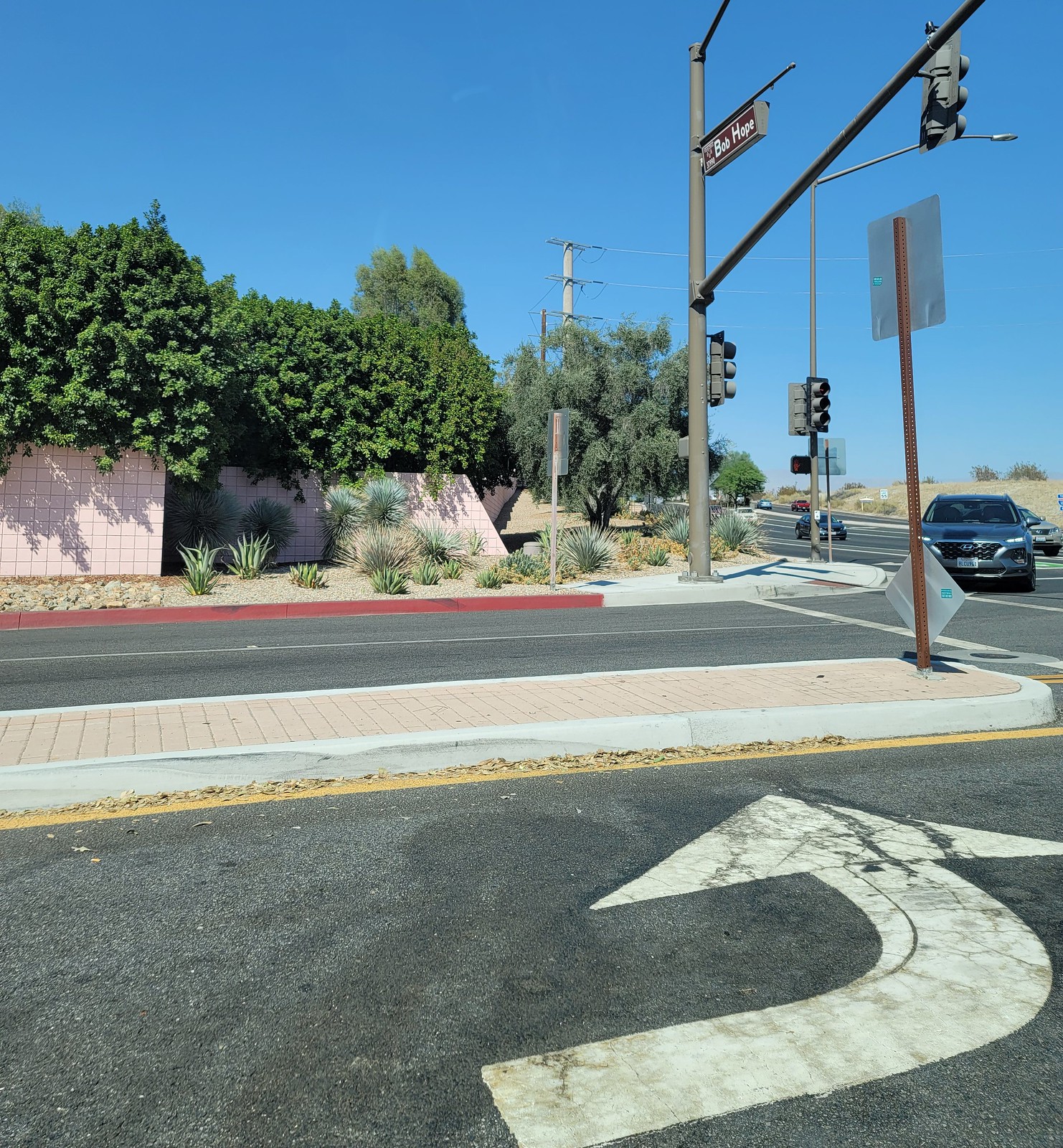A dual carriageway road leads up to a scenic beachfront, as viewed from the right side of the road. A central reservation consisting of a raised pavement features pinkish brick tiles bordered with grey and white concrete edges. The tarmac road is marked with various spills, stains, and shadow patterns, likely from sun exposure. A white directional arrow indicating a left turn is clearly visible on the road surface.

A large people carrier vehicle is turning into the road, adding dynamic movement to the scene. In the background, expansive sand dunes are prominently visible, enhancing the coastal atmosphere. Traffic lights are mounted on robust grey posts, ensuring regulated traffic flow.

The roadside is adorned with abundant greenery, including bushy trees that appear both wild and well-maintained. Among the flora, there are several cactus-like succulents thriving on the pavement, potentially part of a small, informal roadside stall. The overall scene is a vibrant blend of natural and urban elements, capturing the essence of a bustling yet picturesque beachfront roadway.